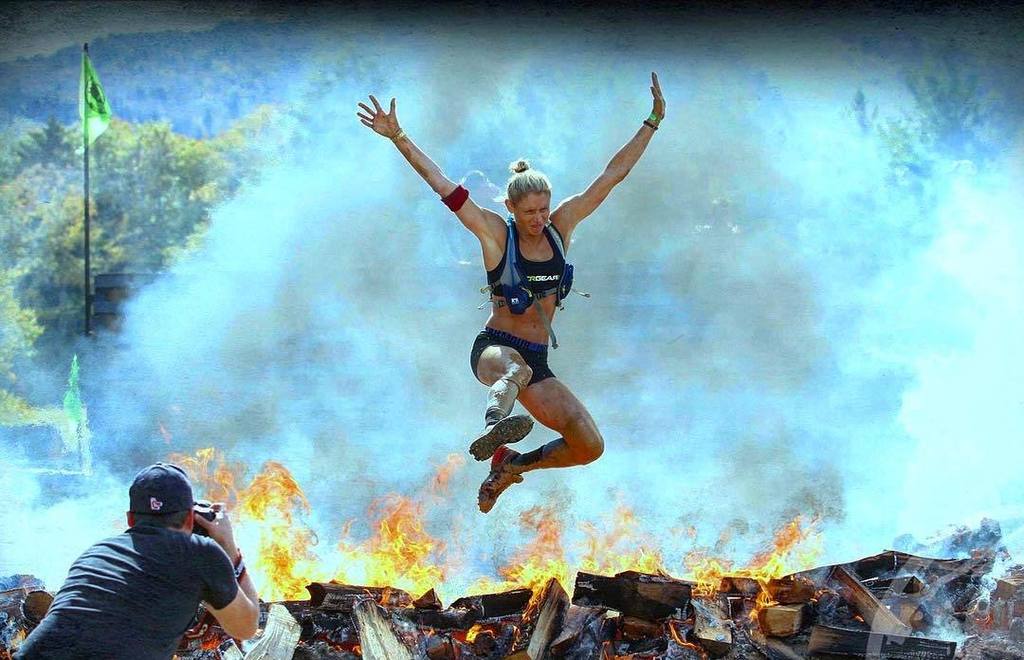The image captures a dramatic scene of a blonde woman, her hair pulled back into a bun, dressed in athletic gear. She is clad in a black sports bra with white writing, paired with blue sports shorts. A red wristband adorns her right arm. She appears to be in mid-air, leaping over a bed of burning debris and flames, with smoke billowing in the background. Her feet are kicked out toward the camera, emphasizing the energy and intensity of the moment. To the bottom left, there is a person captured from behind, squatting down, as they take a photograph. This individual is wearing a black t-shirt and a backward black baseball cap, and is holding a black camera. In the top left corner of the image, a green flag is visible, along with some green trees in the distance, providing a stark contrast to the fiery scene in the foreground. This appears to be an action shot, possibly from a stunt or an adventurous athletic endeavor.